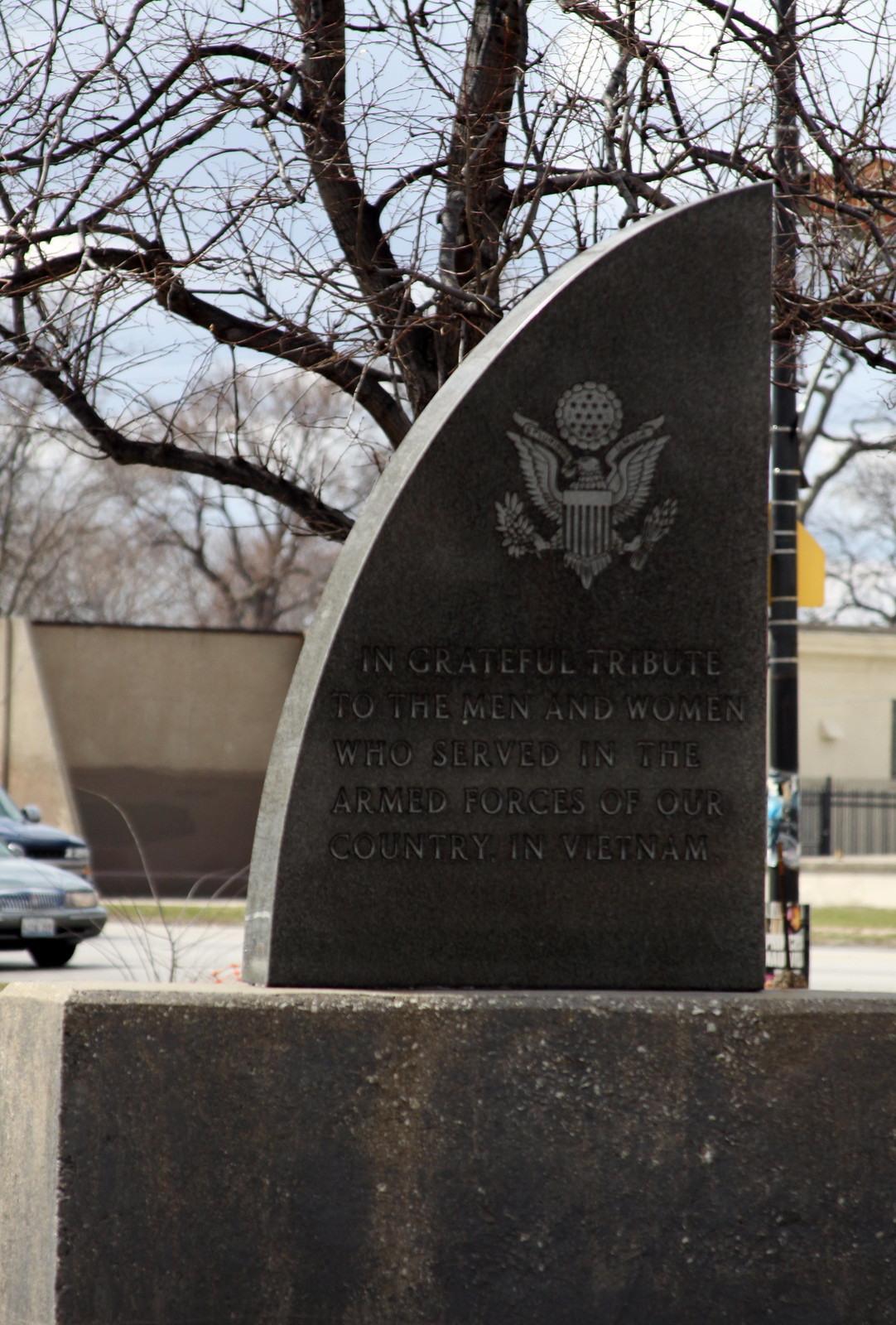The image depicts a detailed Vietnam War memorial made entirely of stone, crafted in the shape of a shark fin with a curved left edge and a straight right edge. This distinct monument rests on a substantial concrete block base. Embellished on the stone is the US government insignia, featuring an eagle clutching arrows and branches amid 13 stars and a banner in its beak. Below the emblem, an inscription reads: "In grateful tribute to the men and women who served in the armed forces of our country in Vietnam." The engravings are set off by the contrast between the darker background concrete and the lighter text. The scene includes a variety of background elements such as a building, a parking lot, trees, and a street light. It's likely a more recent and smaller tribute compared to the main Vietnam War memorial in Washington, D.C. The photo captures the monument in broad daylight with a few clouds dotting the early evening sky.